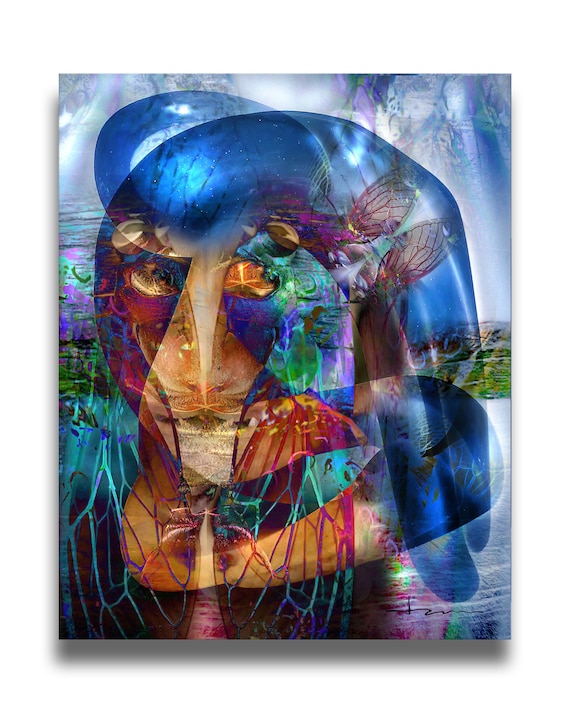The image is an abstract and intricate digital artwork that overlays multiple elements creating a rich and complex visual experience. Dominated by shades of blue, fuchsia, gold, and green, the foreground features a see-through, elongated, balloon-like structure that adds to its surreal quality. Amidst the abstract forms, a semblance of a face with distorted eyes, nose, and mouth emerges, giving a human-like aspect to the composition. To the right, there's a depiction of a lake with concentric circles in the water, hinting at a signature element. The background includes netting in light blue and green hues, resembling wispy grass or vegetation. Vegetative roots and insect wings are interspersed, with locust wings discernible on the left side, adding a touch of nature to the collage. This multifaceted arrangement harmoniously blends hyper-realistic and abstract styles, creating a lexicon of interconnected, layered imagery.